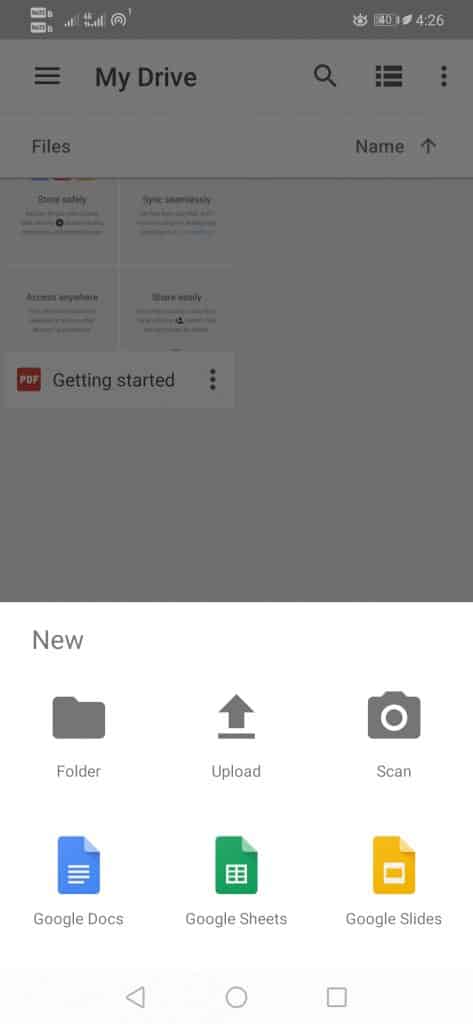The image depicts the interface of Google Drive with various elements visible on the screen. At the very top, there's a grey bar displaying icons such as signal strength, battery life, and time, which reads 4:26. Below this is a toolbar with navigation options, denoted by dashes, lines, and dots.

On the main part of the screen, there's a bright white background. Several icons and file names are visible, including a red square thumbnail for a PDF titled "Getting Started..." and a grey folder labeled "New." Other icons include an upward arrow for uploading files, a camera icon for scanning documents, and several Google application icons: a yellow rectangle for Google Slides, a green sheet for Google Sheets, and a blue document for Google Docs.

The overall layout is clean and organized, displaying the diverse functionalities and file organization within Google Drive.